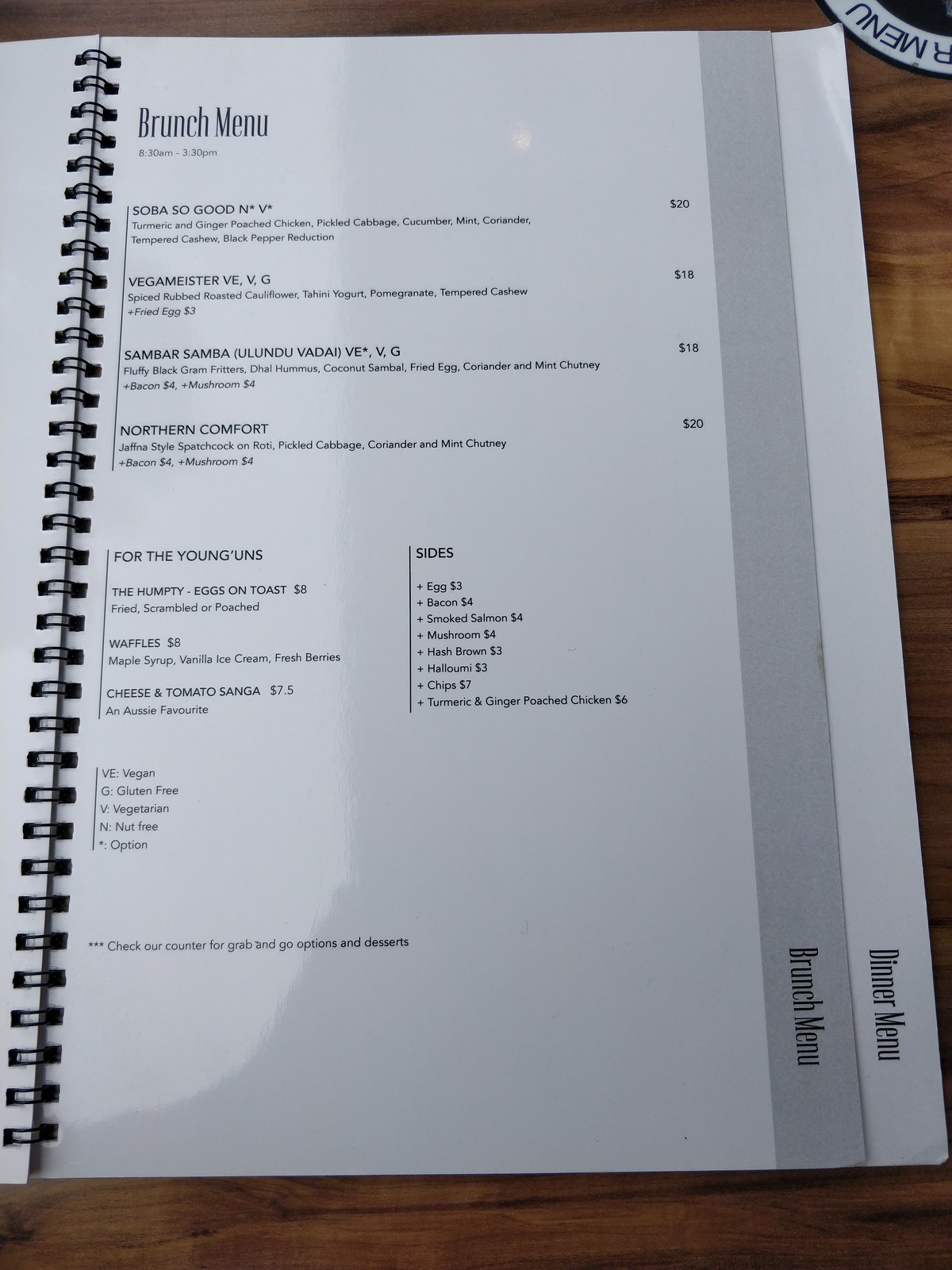**Close-Up of Restaurant Menu on Wooden Table**

In this detailed close-up image, we see a restaurant menu, predominantly displayed against a brown, wooden table. The menu itself, white in color and bound in a spiral notebook format, features text in black and white. The top right corner of the menu is partially covered, revealing a half-circle tab with the letter "R" and the word "Menu" in black letters on a white background.

The visible page is a brunch menu, with additional tabs suggesting the presence of other sections, including a dinner menu. The brunch menu specifies its availability from 8:30 a.m. to 3:30 p.m. At the bottom, three asterisks indicate the availability of grab-and-go options and desserts.

The brunch offerings include:
- **Soba So Good**: Turmeric and ginger poached chicken, pickled cabbage, cucumber, mint, coriander, tempered cashew, black pepper reduction for $20.
- **Vega Meister (VE)**: Spice-rubbed roasted cauliflower, tahini yogurt, pomegranate, tempered cashew for $18.
  
Sides are also available, including:
- **Egg**: $3
- **Bacon**: $4
- **Smoked Salmon**: $4

Other items listed are:
- **Waffles**: $8
- **Cheese and Tomato Sanga**: An Aussie favorite for $7.5

For children, labeled as "for the young'uns," the menu features:
- **Humpty Eggs on Toast**: Available fried, scrambled, or poached for $8, along with other options.

The detailed presentation highlights the menu's variety and provides a glimpse of the dining experience at the restaurant.